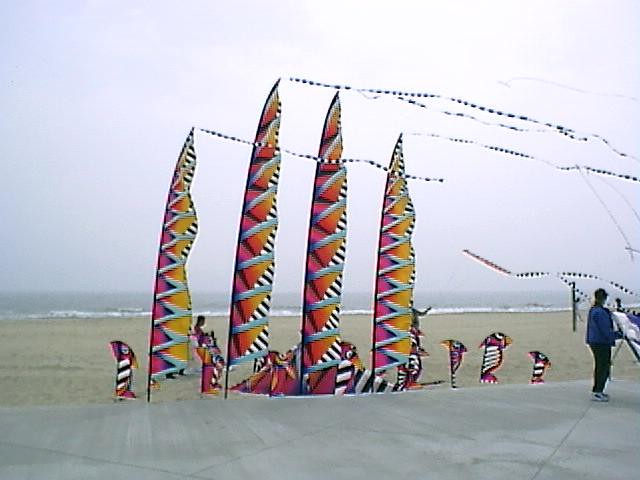This image captures a serene beach scene under a grayish-blue, somewhat illuminated sky, with the sun subtly brightening the horizon. The murky gray waves gently lap at the shore, the white foam emphasizing the soft light brown sand that stretches across the middle of the picture. A concrete walkway can be seen cutting through the front of the image, leading towards the ocean.

In the foreground and stretching along the shoreline are an array of colorful flags mounted on poles. They stand out prominently against the muted backdrop, each adorned with vibrant patterns of pink, purple, blue, and yellow, featuring zigzag stripes and white designs. Some of these flags have long, dark blue and white streamers fluttering in the wind, adding a sense of movement and whimsy. The flags vary in height, with the tallest ones positioned in the middle and smaller ones interspersed between.

Among the flags, a few people can be seen. On the left, a person appears to be seated, possibly on a chair, while another figure stands behind one of the smaller flags, dressed in a blue jacket, black pants, and tennis shoes. The overall scene conveys a peaceful, albeit slightly overcast, day at the beach, with the artistic flags adding a splash of color and life to the tranquil setting.